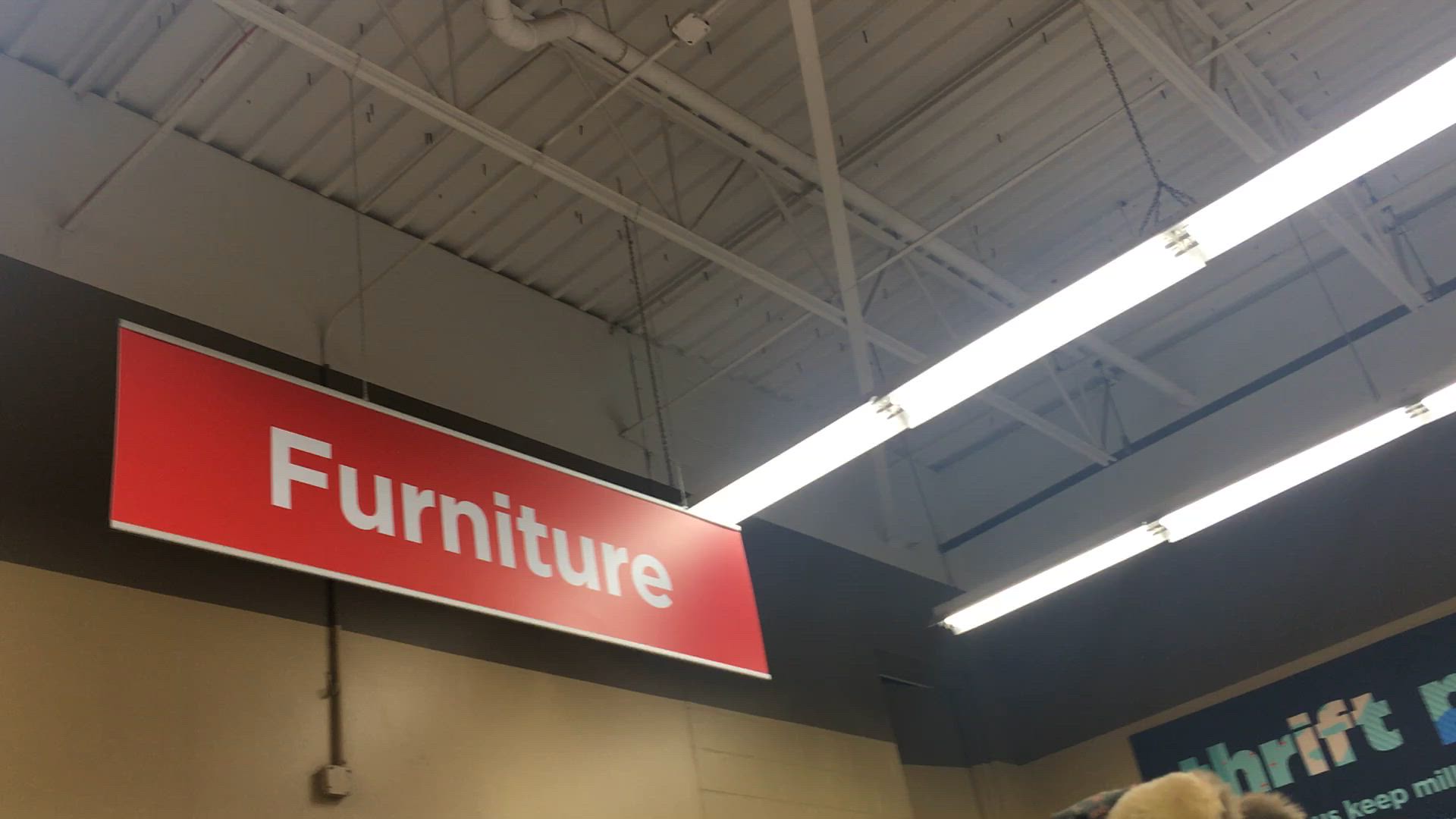The image captures the ceiling of a retail store, featuring an intricate grid of white rails running vertically and horizontally. Integrated within this grid is visible ventilation and a series of white strip lights suspended from black cords, aligned diagonally to the right. In the bottom left corner, a red rectangular sign is affixed to a light brown wall with a dark brown border. The sign prominently displays the word "Furniture" in white font. The bottom right corner of the image reveals the top of a person's light brown hair.